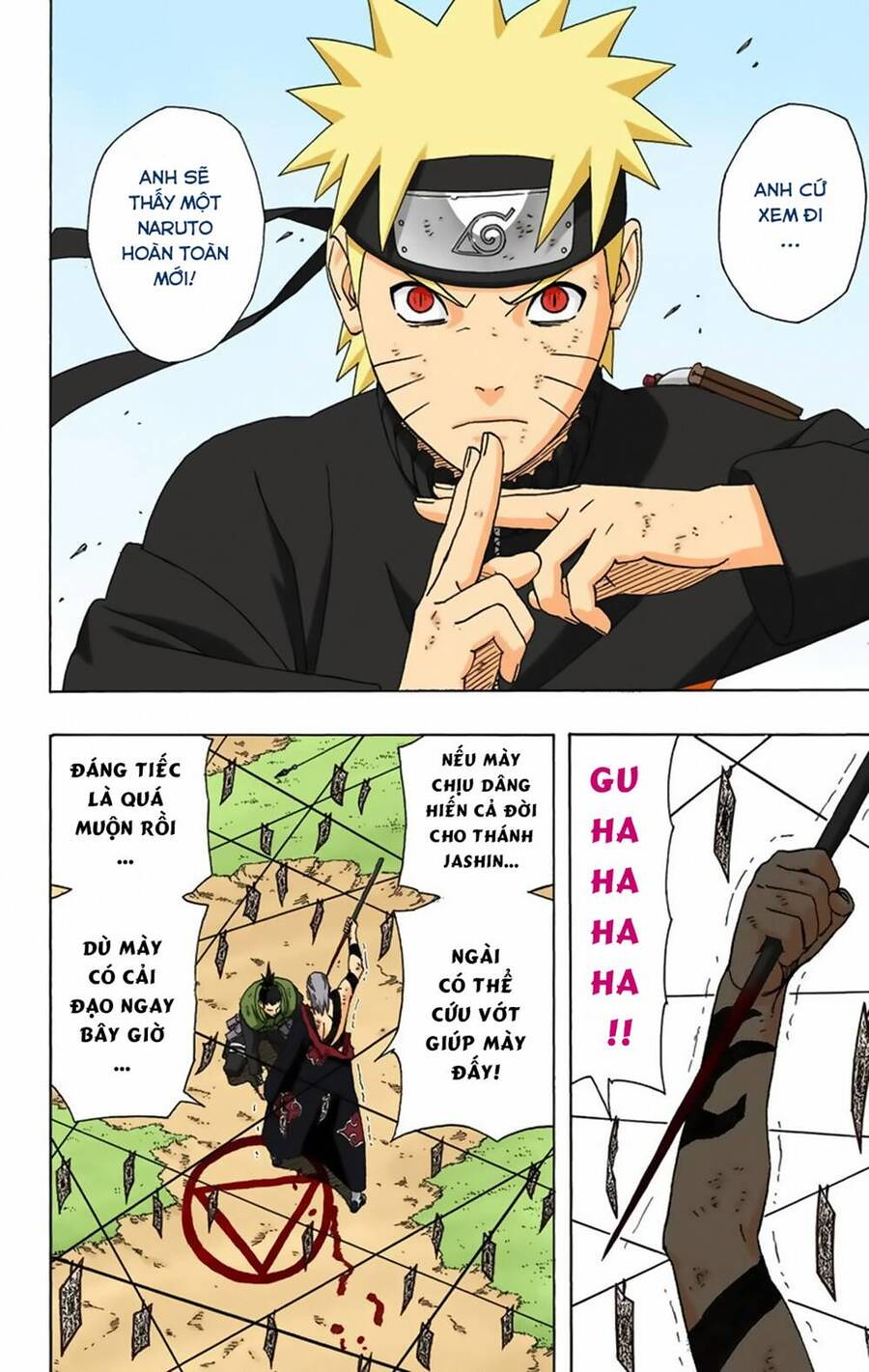The image showcases a Vietnamese comic divided into three distinct sections. The top half of the comic features a single panel depicting a blonde-haired boy with red eyes, wearing a black top and a black headband with silver in front. His hands are positioned as if he's focusing, with fingers crossed in front of him. There are two dialogue bubbles around him featuring Vietnamese text. The scene appears intense, hinting at an imminent action likely involving martial arts.

In the bottom half of the comic, the left larger panel portrays a fierce fight between two men, visibly drawing blood. Vietnamese text is also present, adding a narrative to the brutal altercation. The scene is violent and dynamic, set against a green and brown background with a distinct circle containing a red triangle in it.

The bottom right panel, smaller in size, depicts an arm raised high holding a sharp weapon, possibly a knife or sword. The weapon gleams menacingly, and the action is accompanied by the onomatopoeic text "Gu Ha Ha Ha Ha" in pink, suggesting sinister laughter. This panel conveys a heightened sense of danger and urgency, hinting that the weapon may soon be used in the fight depicted in the adjacent panel.